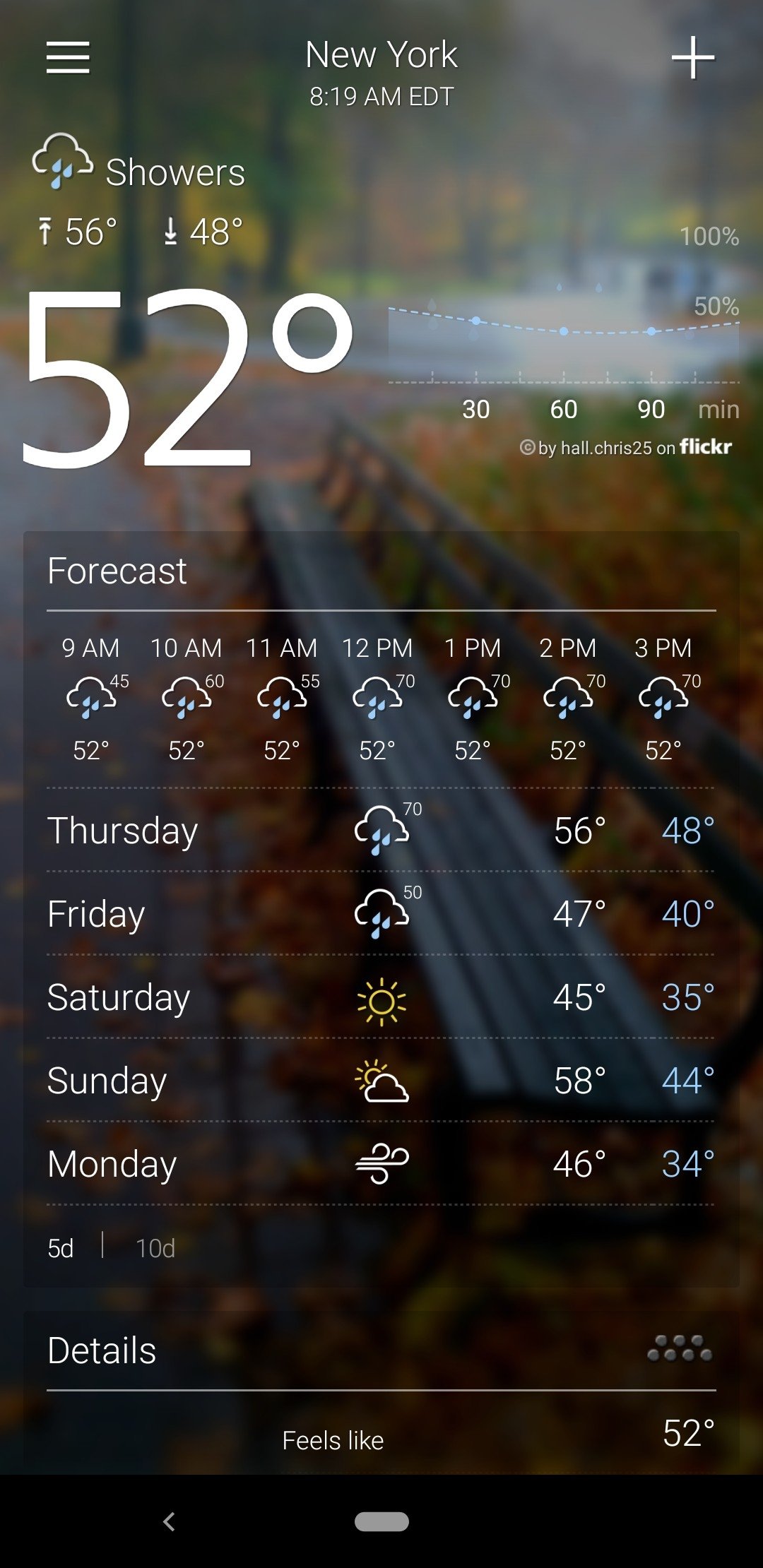This image, captured from a cell phone screen, showcases a serene autumn park scene. The background features a picturesque walking area adorned with fallen leaves in a myriad of fall colors — vibrant oranges and yellows, interspersed with greens and reds. A row of park benches beckons for a respite, while sturdy tree trunks and canopies stretch across the horizon.

Overlaying this tranquil background, white text reads "New York" at the center top, along with a timestamp "8:19 AM EDT." The weather details are prominently displayed on the left side: a cloud icon with raindrops indicates showers, with temperatures showing a high of 56°F (arrow pointing up) and a low of 48°F (arrow pointing down). The current temperature is boldly printed as 52°F. Adjacent to this, a faint bar graph or dot graph illustrates weather data over time, marked with intervals of 30, 60, and 90 minutes and percentages of 100% and 50%.

Below the current temperature, a detailed forecast chart presents further weather information, including pictograms, days of the week, times, and temperature highs. The composition of the image seamlessly blends the natural beauty of the park with the practicality of a weather app display, providing both a visual and informational treat.